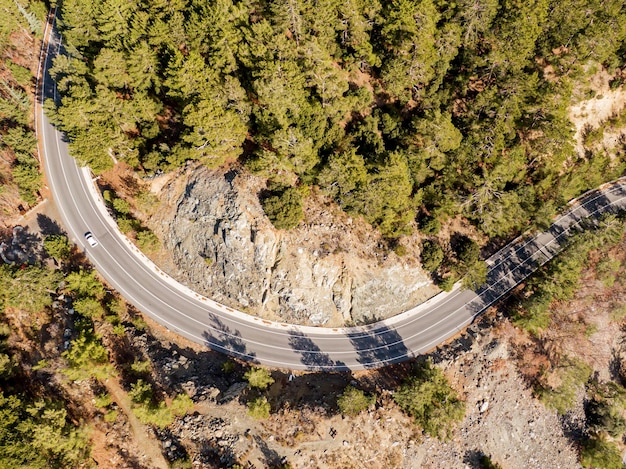This overhead aerial shot captures a curved mountain road snaking through a rugged, rocky landscape. The road, which appears to be a two-lane, possibly European route, is bordered by dense green forest, with tall trees extending their shadows over the black asphalt. Midway through the winding section, a single white car travels on the left side, suggesting it might be in a country with left-hand traffic. The rocky terrain reveals areas where the mountain has been blasted to accommodate the road, exposing black and gray stone faces. The bright, sunny day accentuates the contrast between the greenery of the forest and the starkness of the rocky mountainside, creating a scene reminiscent of a high-end car commercial. The vantage point, several hundred feet in the air, provides a clear view of the landscape's natural beauty and the road's integration into this rugged environment.